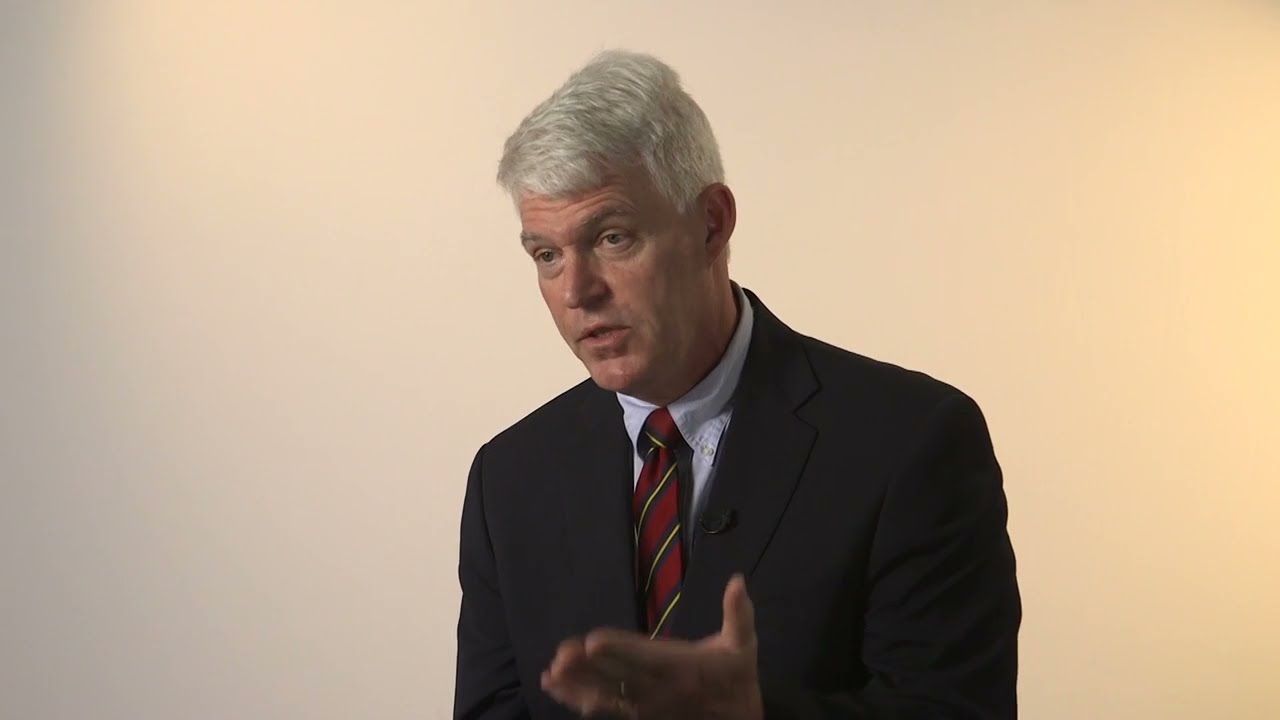In the foreground of a photo with a very light orange or peach background, a middle-aged to older white man, likely in his mid-50s to 60s, is depicted. He has white hair, which is shorter on the sides and longer on the top, neatly combed to the side. His complexion is suntanned, with a reddish hue, and he has visible lines on his forehead along with slight bags under his eyes. The man is wearing a black suit coat over a light-colored shirt, which might be white or light blue, paired with a distinctive red tie featuring blue, yellow, and black diagonal stripes. He appears to be engaged in conversation, possibly being interviewed, as indicated by his concerned expression and the slight opening of his mouth mid-sentence. His gaze is directed upward and to the left, and a microphone is clipped to the right side of his suit, further suggesting he's speaking to someone off-camera. The right side of his face is slightly shadowed, adding depth to his serious demeanor.